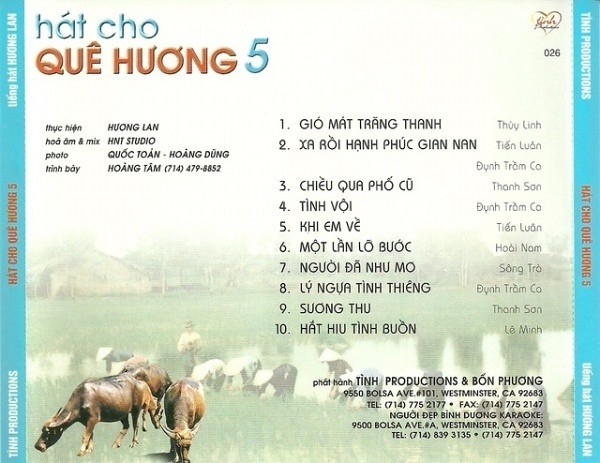This detailed image appears to be the back cover of a Vietnamese music CD titled "HAT CHO KHONG QUE HUONG 5." The square image is bordered vertically on both sides with blue bands, featuring white text on the top and bottom with red text in the center. The background showcases a light gray sky with houses, trees, and grass at the bottom, along with a pond. In the lower left corner are two tan bulls with long horns. In the lower right corner, there is black, right-aligned text that provides an address, phone, and fax number for 10 Productions, located at 9550 Bolsa Avenue, Suite 101, Westminster, California, 92683.

The CD’s central artwork includes a man walking through a rice paddy field, surrounded by people wearing white hats and black outfits, presumably harvesting rice. The man is amidst light brown cattle. At the top left of the image, it prominently displays the title "HOTCHO" in blue letters, followed by "KHONG QUE HUONG" written in all caps red letters, and a blue number "5" to the right of this text.

Below the title, the CD tracklist is presented in two left-aligned columns, listing ten tracks numbered one to ten vertically on the right side, with each number accompanied by black text in Vietnamese, likely denoting the song titles and artists.